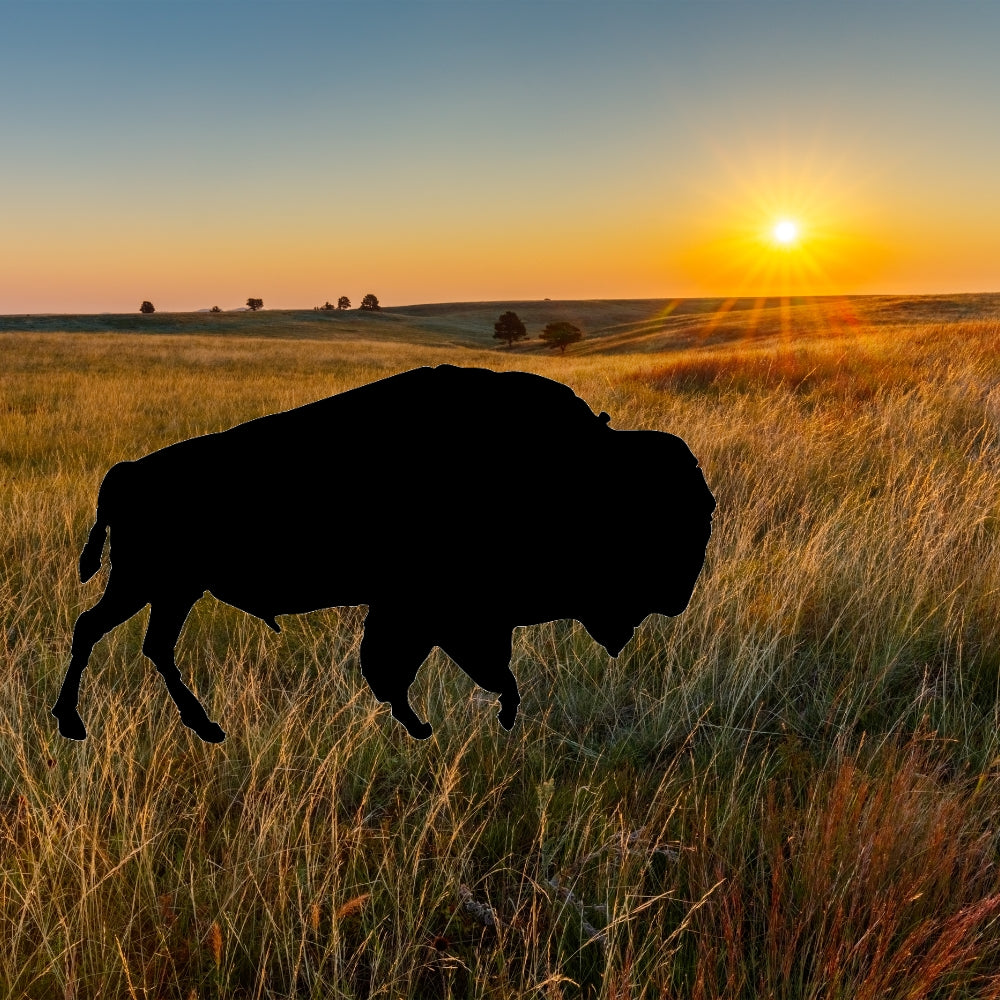In this edited photograph, a vast prairie field extends into the horizon under a light blue sky that transitions to orange near the bottom, suggesting the time is dusk as the sun sets in the right corner of the image. The prairie is covered with tall, brown and green grasses that seem to waver in the gentle wind. In the distance, various green-leaved trees are scattered across the gently rolling landscape. The foreground features an artistic overlay: an outlined silhouette of a buffalo, likely digitally added to evoke the absence of the once-present animal in this ecosystem. The silhouette stands out starkly with its black interior and white border, contrasting with the natural beauty of the prairie scene.